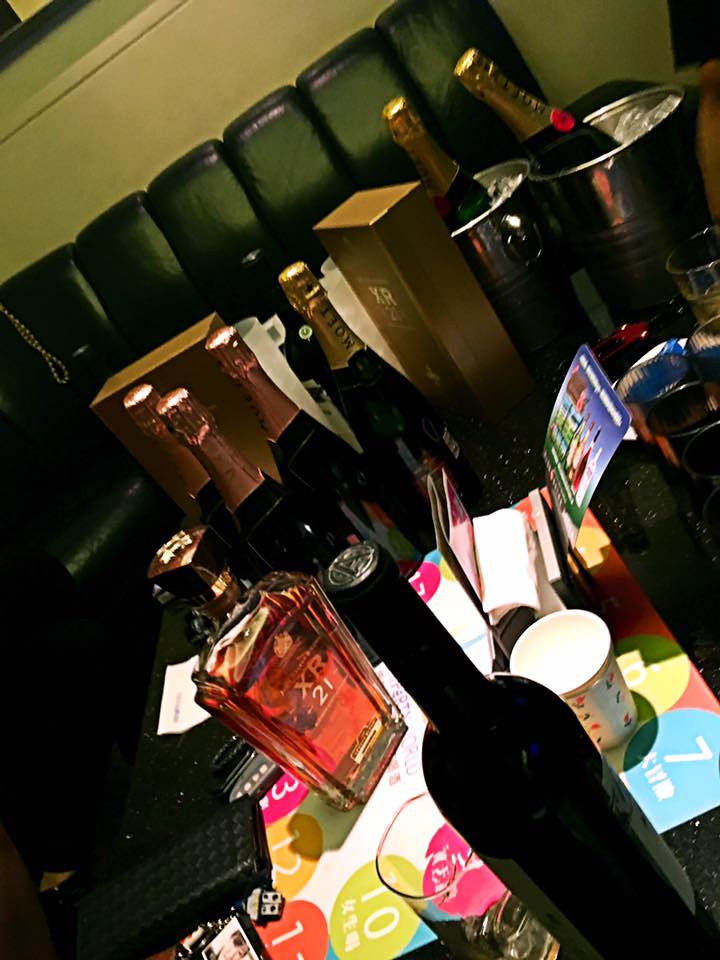This photograph captures a disarray of alcohol bottles spread across a dimly lit party table in front of a black, tufted leather booth. The assortment includes unopened bottles of champagne with gold foil tops nestled in ice-filled buckets, alongside other various unopened liquors such as a unique pinkish bottle marked "XR 21" in a cut-crystal design. A black wine bottle with matching foil is prominently placed in the foreground. The tabletop is cluttered with an assortment of items including drinking glasses, paper cups, napkin holders, and a party card with graphics. There's also a possibility of a wallet or cell phone case among the scattered objects. The lighting casts a reflective glow from above, bouncing off the foil tops and creating a dark ambience that suggests the party has not yet begun. Additional details such as a high-backed booth with tufted, black cushions and a somewhat angled perspective looking down the table add to the scene’s chaotic yet festive atmosphere.